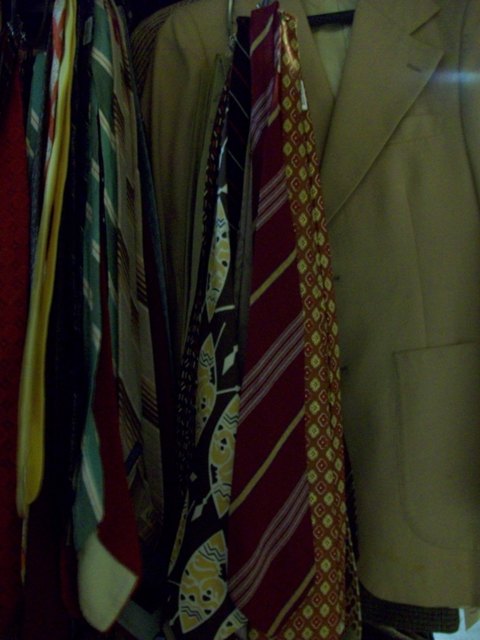This dimly lit close-up photograph captures a section of a closet brimming with a variety of clothes, predominantly showcasing a vibrant array of ties. On the left, a brown coat with a white inner lining subtly peeks into the frame, suggesting an assortment of apparel beyond the visible ties. The ties themselves are a cacophony of colors and patterns: one tie on the left features a striking blend of red with yellow diamonds, while another showcases black adorned with yellow and white symbols. Central to the image, a red tie with two sets of three white stripes and a yellow stripe in between stands out. Additional ties display hues of orange, blue, green, white, beige, and even floral designs, hanging meticulously off what appears to be a ring-like hanger. In the background, blurred yet discernible, are a few suit jackets that reinforce the sense of organized yet bountiful wardrobe space.